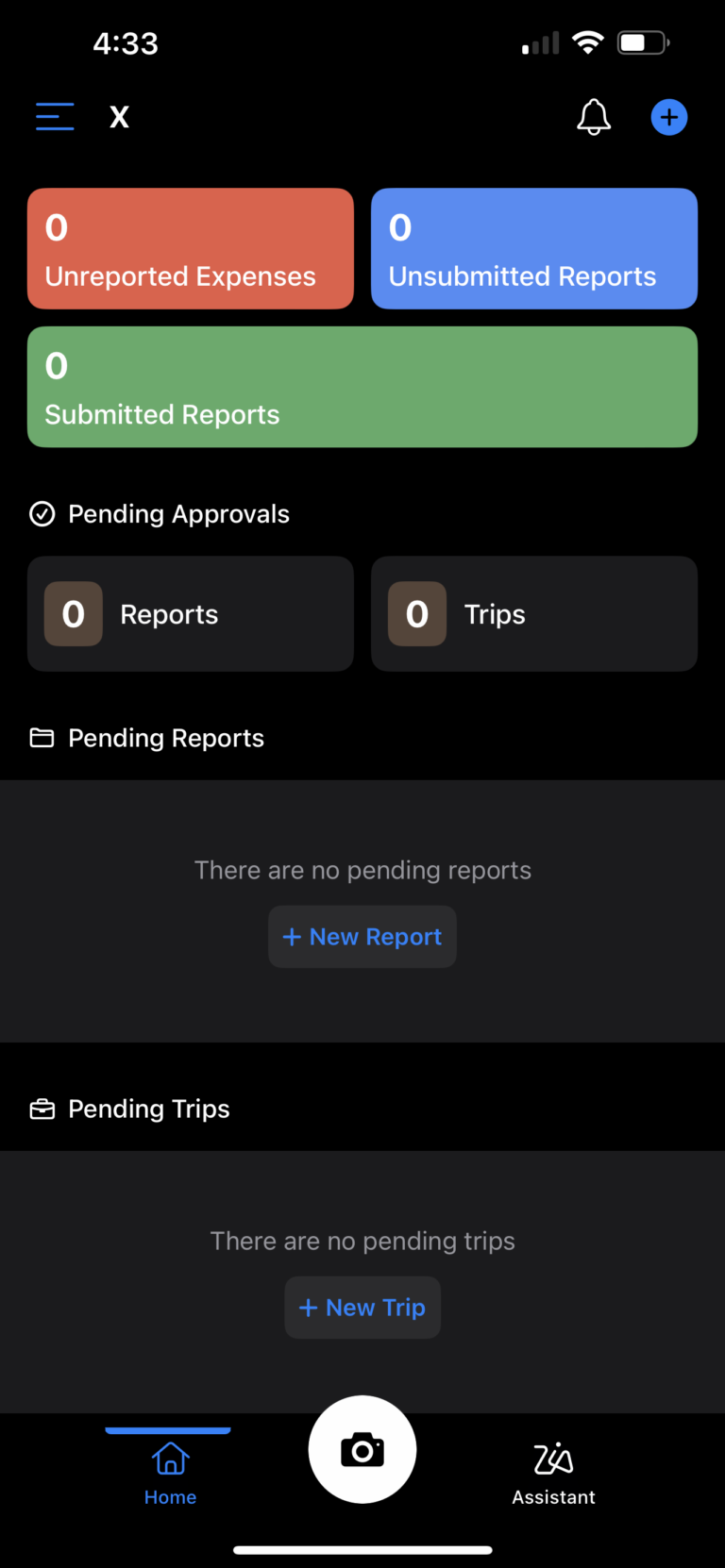This detailed screenshot, likely captured on a tablet or smartphone, displays an app interface focused on managing reports and trips. At the top left, the time is shown as 4:33 (unspecified AM or PM). On the top right, icons indicate a weak signal with only one lit rectangle, followed by a wireless signal icon, and a partially filled, overturned battery icon. Three blue lines sit adjacent to a white ‘X’ symbol. Further right, there is a notification bell and a circle containing a black plus sign.

Below the top bar, an orange rectangle displays a white zero, indicating no unreported expenses. To its right, two labeled sections, "Unsupported Reports" and "Submitted Reports," both show a zero count, represented within a green rectangle containing white text.

In the interface's black section beneath, a circle with a white checkmark labeled "Pending Approvals" is visible. There are two dark gray boxes with small, rounded brown squares inside. The first box on the left, labeled "Reports," shows zero, and the one on the right, labeled "Trips," also displays zero. Adjacent to these, a folder labeled "Pending Reports" in white text appears.

A space separates this from a dark gray or lighter black rectangle stating, "There are no pending reports" in dark gray text. A button in lighter black with blue text reads, "+ New Report." Below, a section labeled "Pending Tips" with a briefcase icon in white text is shown. Similarly, a lighter black rectangle with dark gray text reads, "There are no pending trips," followed by another off-black rectangle with blue text labeled, "+ New Trip."